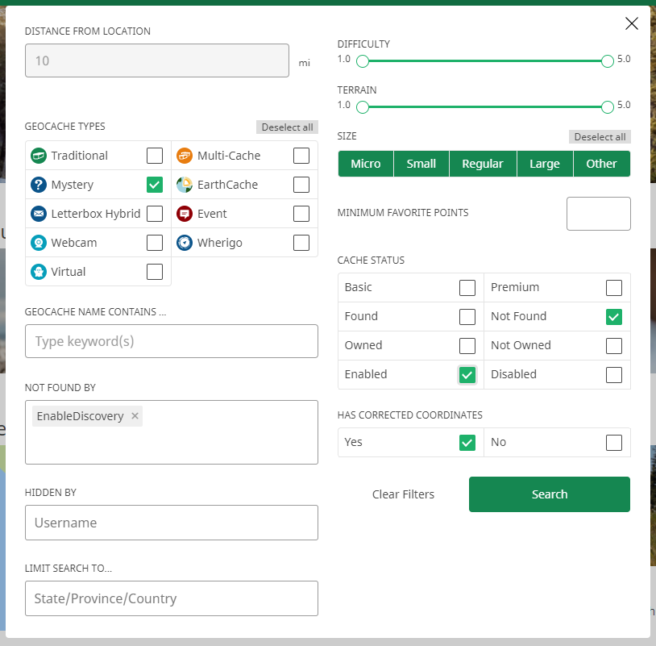The photograph captures a webpage featuring a dominant white pop-up box that takes up most of the screen. The webpage background visible behind the box exhibits shades of green, brown, and blue. The pop-up displays a user interface for geocache search options. Under the "Distance from Location" heading, the user has entered "10 miles."

The pop-up includes green bars indicating difficulty and terrain levels, both ranging from 1 to 5. On the left side, the section titled "Geocache Types" features several icons with different cache categories:

1. Traditional - Green circle
2. Mystery - Blue circle with a question mark
3. Letterbox Hybrid - Blue circle with an envelope
4. Webcam - White webcam icon
5. Virtual - Blue circle with a ghost
6. Multi-cache - Orange icon
7. EarthCache - Earth icon
8. Event - Icon similar to a calendar
9. Where I Go - Icon for navigational game cache

Additional filters are available for specifying geocache name, keywords, and the status of caches not found by the user. Other options include enabling discovery mode, filtering caches hidden by a specific username, limiting searches to a state/province/country, setting a minimum number of favorite points, and specifying cache statuses. The user has selected options for enabled caches and those not yet found.